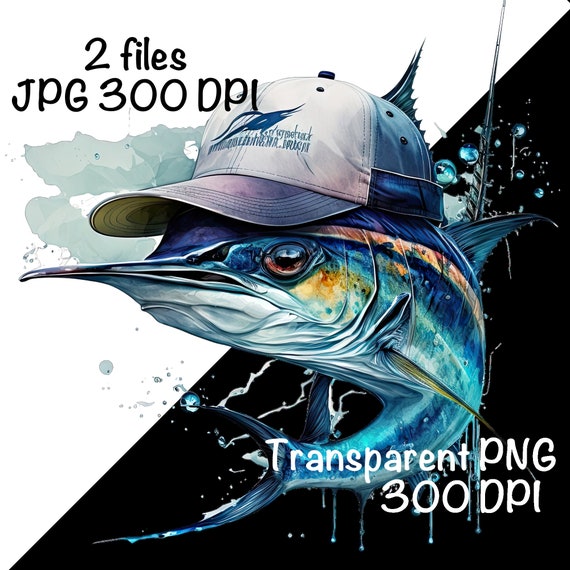The image appears to be an advertisement for a graphic designer, featuring a highly stylized digital representation of a marlin or swordfish. The marlin is depicted in dynamic motion, with its body arched and tail swishing in one direction while its pronounced bill extends in the opposite direction. It sports a colorful baseball cap adorned with a solid blue graphic of another fish and some indiscernible lettering. The fish itself exhibits a vivid palette of blue, yellow, and pink hues, alongside a striking reddish eye. The background is split diagonally into two triangles: the top half is predominantly white with subtle blue swirls, while the bottom half is a stark black filled with floating blue bubbles. Overlaying the image are file type labels — "JPEG 300 DPI" at the top and "Transparent PNG 300 DPI" at the bottom — emphasizing the digital nature of the artwork.